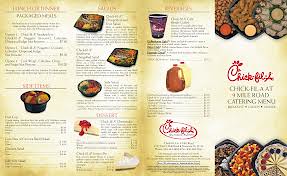The image depicts a Chick-fil-A menu catering spread, albeit somewhat blurry and difficult to read due to maximum zoom. In the upper left corner, there is some text followed by an image of a bowl containing food beneath it with additional text below this bowl. 

To the right, three bowls filled with different food items are shown at the top, each accompanied by descriptive text. At the bottom, there is an image featuring two slices of pie with text adjacent to it. Next to the pie image, a cup is pictured with text beside and beneath it. Below the cup, there are gallon containers of tea and lemonade, each with corresponding text.

Towards the bottom left, the iconic Chick-fil-A logo is displayed with more text underneath it. The far right corner of the image shows the front cover of the menu. The top section of this cover features more bowls of food. Centralized at the bottom of this menu cover, the text reads "Chick-fil-A 9 Mile Road Catering Menu."